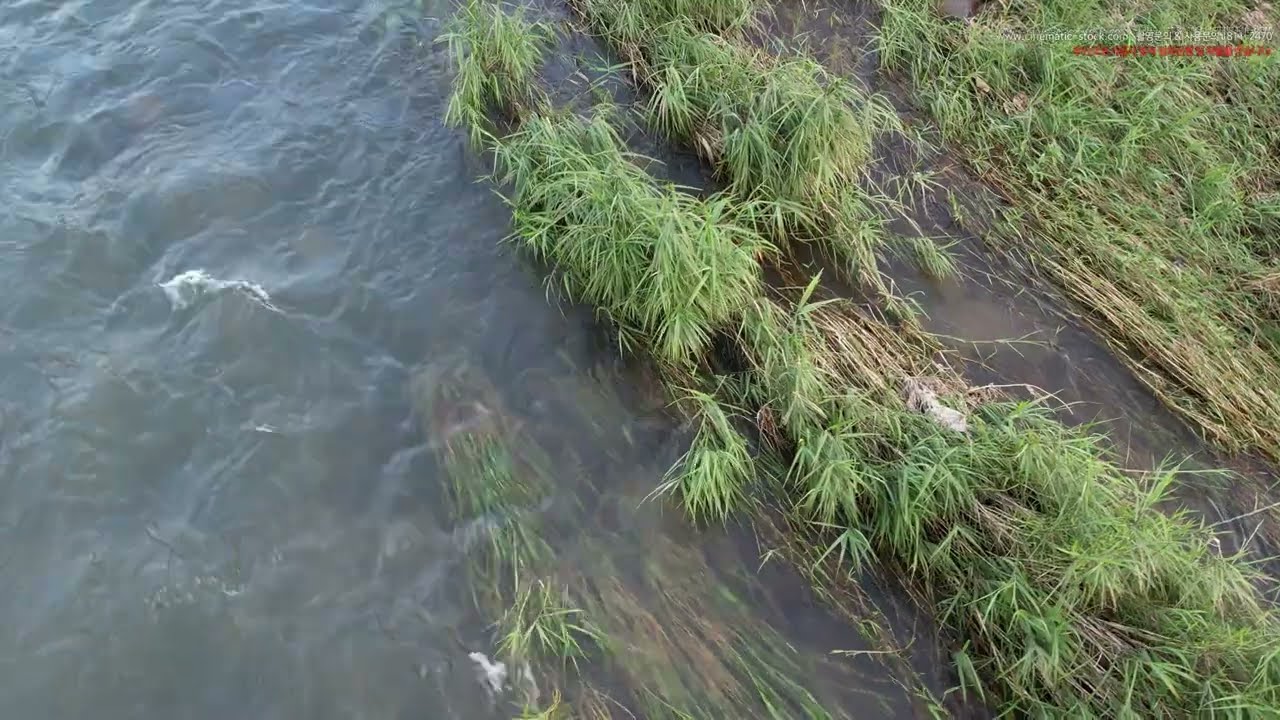An overhead shot captured from about 10 feet above a leisurely flowing river or stream, possibly using a drone. The river meanders through patches of grass and weeds, suggesting slight flooding or overflow onto the grassy banks. The water is light greenish in hue, and despite its modest size, it holds some small, fast-moving waves with white caps. Beneath its clear surface, stones of varying sizes, some as large as 4 to 5 feet in diameter, are visible amongst the vegetation. The greenery includes both lush green leaves and dried, tannish-brown ones, indicative of hot weather conditions. The flow is stronger towards the middle but slows as it approaches the shoreline on the right. Small grass and vegetation submerged in the water are seen bending under the current. Text in white and red letters appears faintly in the top right corner of the image, although it is difficult to read.